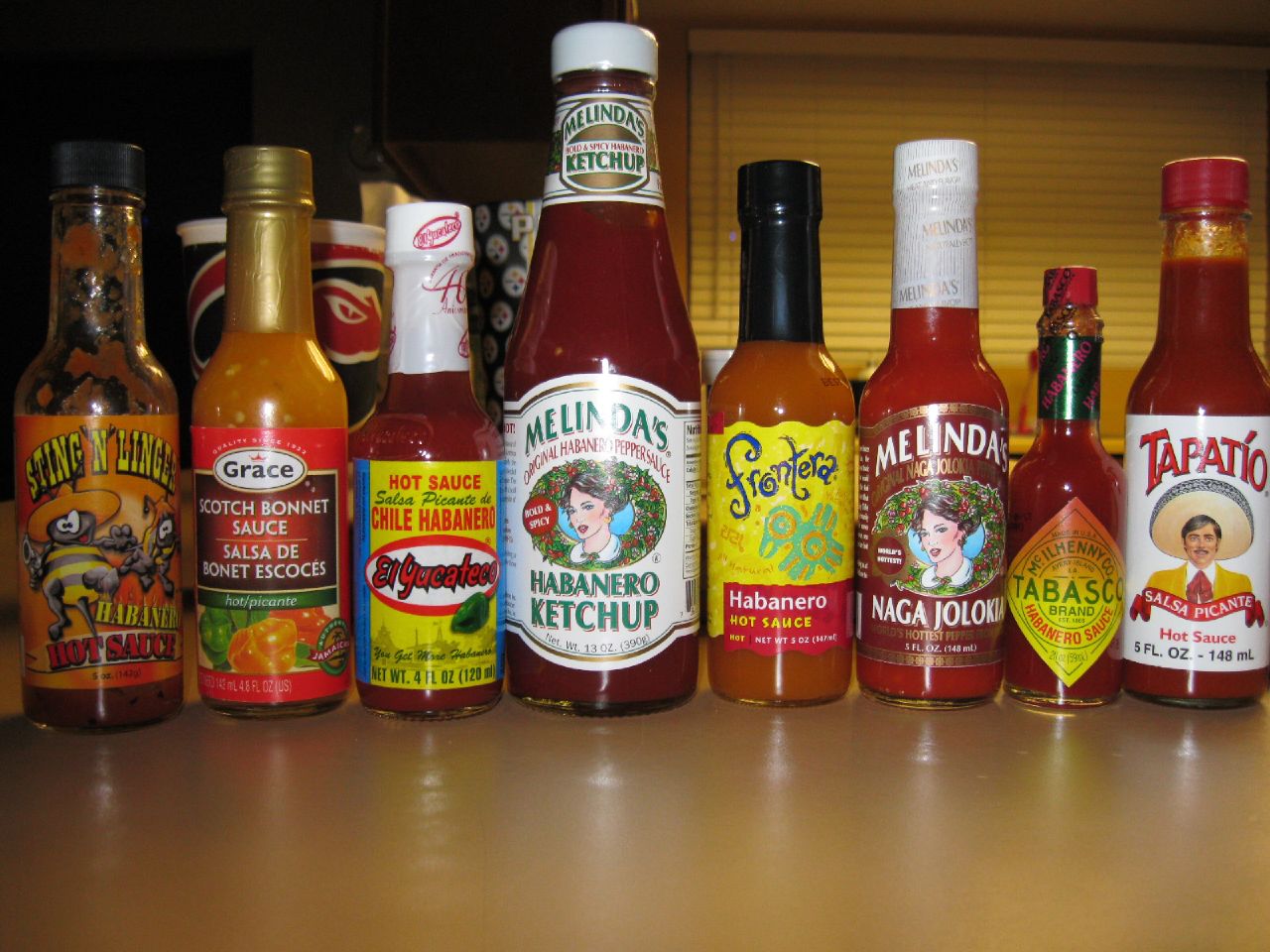The photograph captures a colorful assortment of eight different hot sauce bottles set on a light tan countertop. The array includes a variety of brands and flavors, each with distinct and vibrant labels. From left to right, the hot sauces are:

1. **Sting and Linger Hot Sauce** - this bottle prominently features red in its label.
2. **Grace Scotch Bonnet Sauce (Salsa de Bonnet Escoches)** - this orange sauce stands out with its red label.
3. **El Yucateco Hot Sauce, Chili Habanero** - bearing a yellow and blue label, this bottle is smaller in size compared to others.
4. **Melinda's Habanero Ketchup** - the largest bottle, it's centrally located with a white label and a white cap.
5. **Frontera Habanero Hot Sauce** - characterized by a yellow label and black wrapping.
6. **Melinda's Naga Jolokia Sauce** - another Melinda's variety, this bottle features an orange label and a black cap.
7. **Tabasco Brand Habanero Sauce** - a smaller bottle with a yellow label which appears unopened.
8. **Tapatio Salsa Picante Hot Sauce** - positioned at the far right, it has a white label and a red top.

In the background, the scene is framed by closed, pleated window blinds that lend a yellowish light to the setting. The countertop beneath the bottles is uniformly light brown, drawing focus to the vivid array of hot sauces. The photograph offers a close-up view, emphasizing the texture and color variations among the bottles.